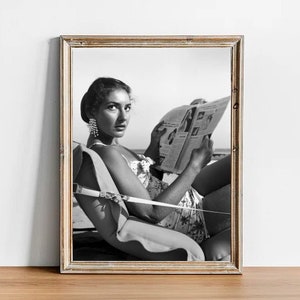The photograph shows a framed black and white portrait of a woman, presented on a semi-gloss wooden table with a moderate brown hue. The frame is old and weathered, featuring remnants of white paint that suggest a past life of more vibrant color, now subdued by time. The frame has a few nicks and scratches, adding to its vintage character. The image within depicts a woman lounging in a cabana chair, positioned on a large cushion. She wears a white one-piece swimsuit adorned with a floral pattern, indicative of an old-fashioned style, and her dark hair is tied back in a bun. Accentuating her elegant look are long, fancy diamond earrings. The woman is immersed in reading a magazine, holding it with both hands while her body slightly twists to peer over her shoulder towards the viewer. Soft daylight suggests she might be outdoors, possibly at a beach, with faint hints of sand and water. The framed photograph leans against an off-white wall, contrasting subtly with the light tan, almost sandy, wooden floor it rests upon. The overall ambiance evokes a nostalgic and serene moment, captured in mid-20th century leisure.